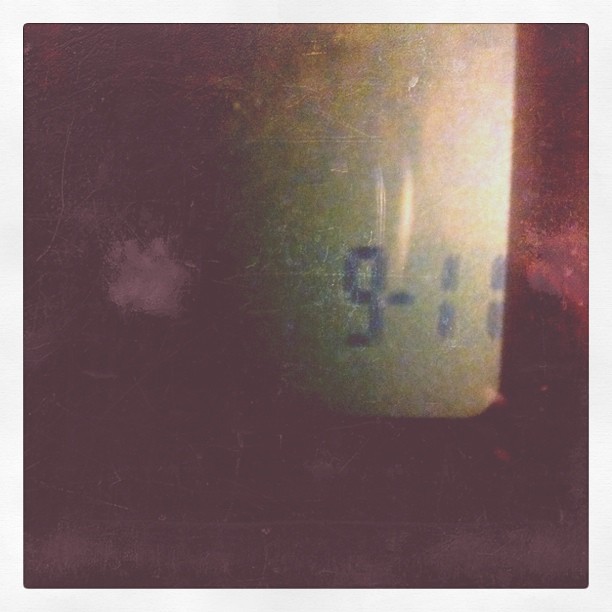The image features a largely purple background with a streak of lighter purple and a splotch of white near the center-left. Dominating the center of the image is a cylindrical object that transitions from green at its bottom to yellow toward the top. This object appears scratched, rusted, and worn, giving it a beat-up appearance. Imprinted at the bottom of the cylindrical item is the number "9-11" in a black, digital clock-style font, with the number '1' notably split in the middle. The photo has a simple composition with only a few colors—primarily shades of purple, green, yellow, and black digits. There is no additional text or imagery aside from these elements, creating a stark yet contemplative scene that evokes curiosity and perhaps a somber tone.